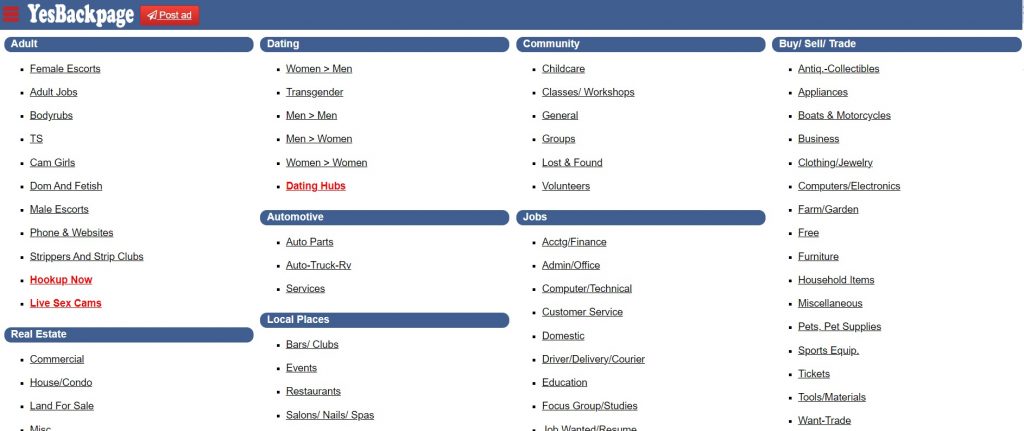In the image, you see a screenshot of the website Yes Backpage, which resembles a Craigslist-style classified ads platform. 

At the very top, a blue border frames the page. In the upper left corner, a red drop-down menu is indicated by three horizontal red lines stacked on top of each other. Directly to the right, the logo "Yes Backpage" is prominently displayed, followed by a red button labeled "Post Ad" in white text.

The rest of the page has a clean, white background with various categories laid out in a structured format. Each category is presented in a long, skinny rectangle with rounded corners and a colored background.

The first category, titled "Adult," is highlighted in blue with white text and includes several bullet points in black, listing:
- Female Escorts
- Adult Jobs
- Body Rubs
- TS (Transsexual)
- Cam Girls
- BDSM and Fetish
- Male Escorts
- Phone and Websites
- Strippers and Strip Clubs
- Hook Up Now (in red)
- Live Sex Cams (in red)

Below this, the "Real Estate" category is displayed with bullet points for:
- Commercial
- House/Condo
- Land for Sale
- Miscellaneous

To the right, another column starts with the "Dating" category, listing options such as:
- Women > Men
- Transgender
- Men > Men
- Men > Women
- Women > Women
- Dating Hubs (in red)

Following that is the "Automotive" category, with bullet points for:
- Auto Parts
- Auto, Truck, RV Services

Next, the "Local Places" category lists:
- Bars/Clubs
- Events
- Restaurants
- Salons/Spas

In the adjacent column to the right, the "Community" category includes:
- Child Care
- Classes/Workshops
- General Groups
- Lost and Found
- Volunteers

Underneath this is the "Jobs" category, featuring:
- Accounting
- Accounting/Finance
- Admin/Office
- Computer/Technical
- Customer Service
- Domestic
- Driver/Delivery/Courier
- Education
- Focus Group/Study
- Job Wanted/Resume (this entry is cut off at the bottom of the page)

Finally, the last column on the right begins with the "Buy/Sell/Trade" category, which includes:
- Antiques/Collectibles
- Appliances
- Boats and Motorcycles
- Business
- Clothing and Jewelry
- Computers/Electronics
- Farm/Garden
- Free
- Furniture
- Household Items
- Miscellaneous
- Pets
- Pet Supplies
- Sports Equipment
- Tickets
- Tools/Materials
- Want/Trade

The categories and their respective subheadings are neatly organized, making it easy to navigate through the wide array of available sections on the Yes Backpage site.